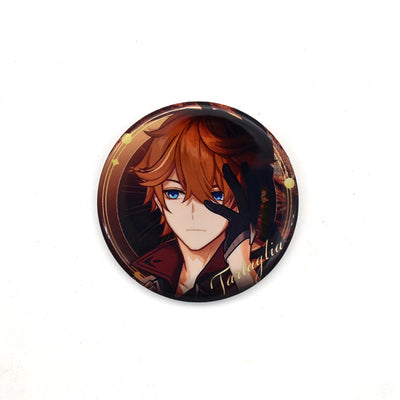The image depicts a round pin or button featuring an anime character with the name "Tartaglia" inscribed in script on the lower right portion. The character has tousled, reddish-brown hair that flops over his piercing blue eyes with long, sweeping messy bangs, and shorter hair on the sides. His striking blue eyes are keenly noticeable above his angular chin and thin nose. He exhibits a straight-faced expression and wears a partially visible black glove on the hand he's holding up to his fair-skinned face. Tartaglia is dressed in an open-collared maroon jacket. The background within the circular frame showcases a dark brown to golden hue with some faint yellow borders adorned by orbs and stars, enhancing the composition. The overall design, suggestive of Japanese anime or manga style, is clearly intended for fans who might wear it to show their admiration for the character.